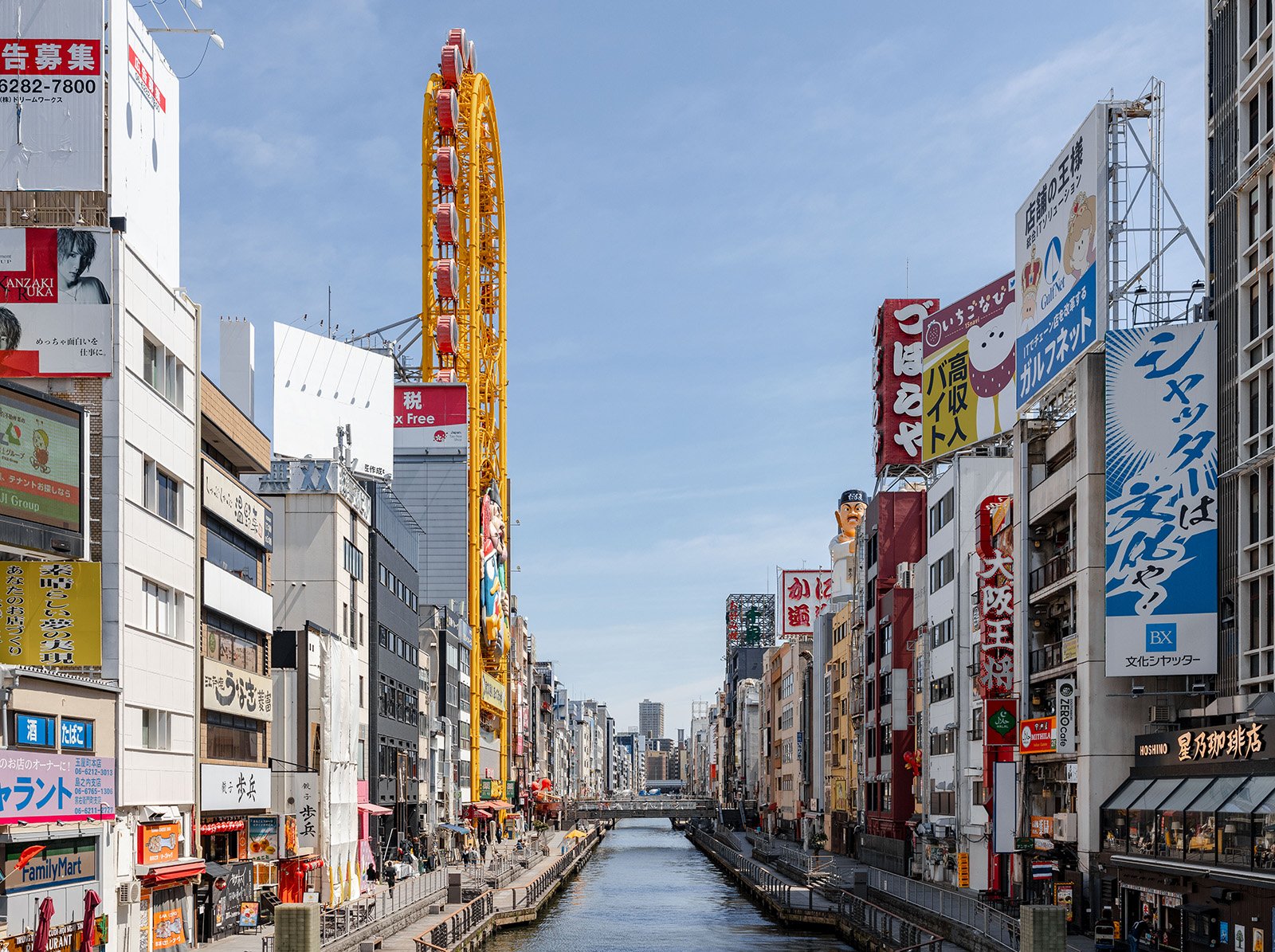The image depicts a bustling, densely populated Asian city, potentially in China or Japan, characterized by a large channel of water running through its center. A bridge spans the river in the distance, providing a connection between the two sides of the city. Lining both banks of the river are tall buildings, vibrant with diverse colors such as white, blue, red, gray, and orange, that suggest a mix of restaurants, storefronts, and possibly apartments. Many of these buildings feature signs and billboards adorned with Chinese or Japanese characters.

On the left side of the river, a massive Ferris wheel stands out with its yellow frame and red passenger cars, towering above the adjacent buildings. At the edge of the river, people are seen walking along gray cement walkways, bordered by metal railings, indicating a busy, urban lifestyle. The scene is rich in detail and brimming with activity, capturing the essence of a lively metropolitan area.